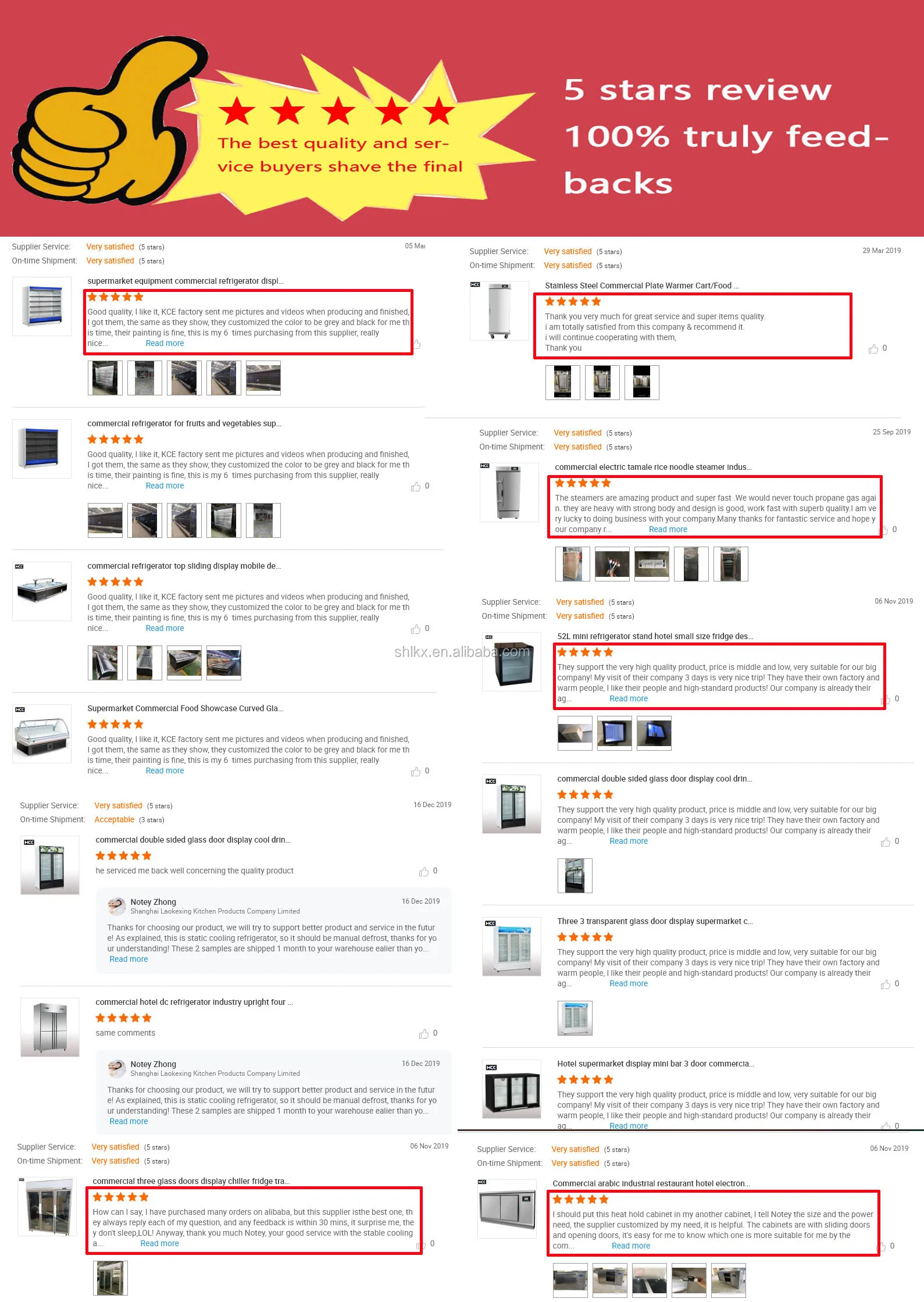The following is an enhanced and detailed caption based on the provided description of an image containing reviews of restaurant equipment.

---

This screenshot displays a series of customer reviews for various types of restaurant equipment, including categories such as sliding glass doors and freezers. Due to the small print, the text, even when enlarged, remains challenging to read clearly.

At the top of the image, a prominent rectangular red banner features multiple elements: 
- On the left side, an animated graphic of a right hand giving a thumbs-up, rendered in gold and outlined in black.
- Next to the animated hand, there is a pointed yellow shape with the following text in red at the center: "The Best Quality in Service Buyers."

Above this text within the yellow area are five red stars. To the right of this section, it reads "Five Stars Review, 100% Truly Feedbacks" in bold white text set against the red background.

Beneath this red banner, the background transitions to white, showcasing approximately 16 categories of restaurant equipment, with eight categories listed on each side (left and right). Each category is accompanied by a small image depicting the respective item of restaurant equipment, followed by corresponding reviews. Among these reviews, six are highlighted with a red outline, indicating their special prominence. Each product has received a five-star rating, as indicated by the star graphics next to each review.

---

This caption provides a clear, detailed, and organized description of the visual content highlighted in the screenshot.